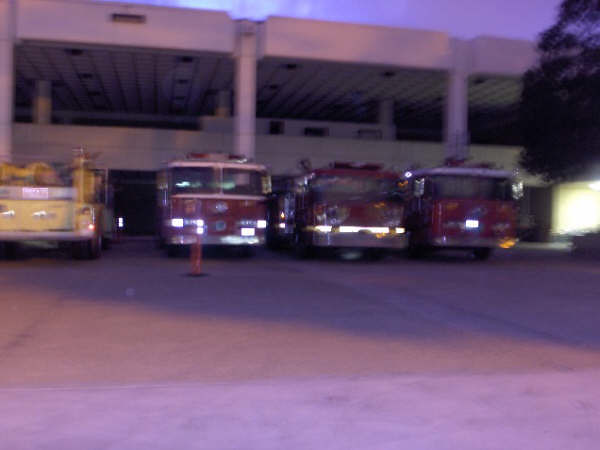This is a very blurry landscape-oriented photograph of a parking lot in front of a white, two-story concrete parking garage. The sky is a dark purple and cloudy, indicating it was taken at twilight. The blurry image shows a line of four emergency vehicles: three red fire trucks facing the camera, partially backed under or just up against the edge of the garage, and one yellow vehicle, possibly an EMT truck, parked facing the opposite direction with its rear towards the camera. An orange traffic cone is visible in front of the second fire truck from the left. On the far right of the picture is a tree, next to the entrance to a building. A small, indistinct sign is also present behind one of the vehicles.